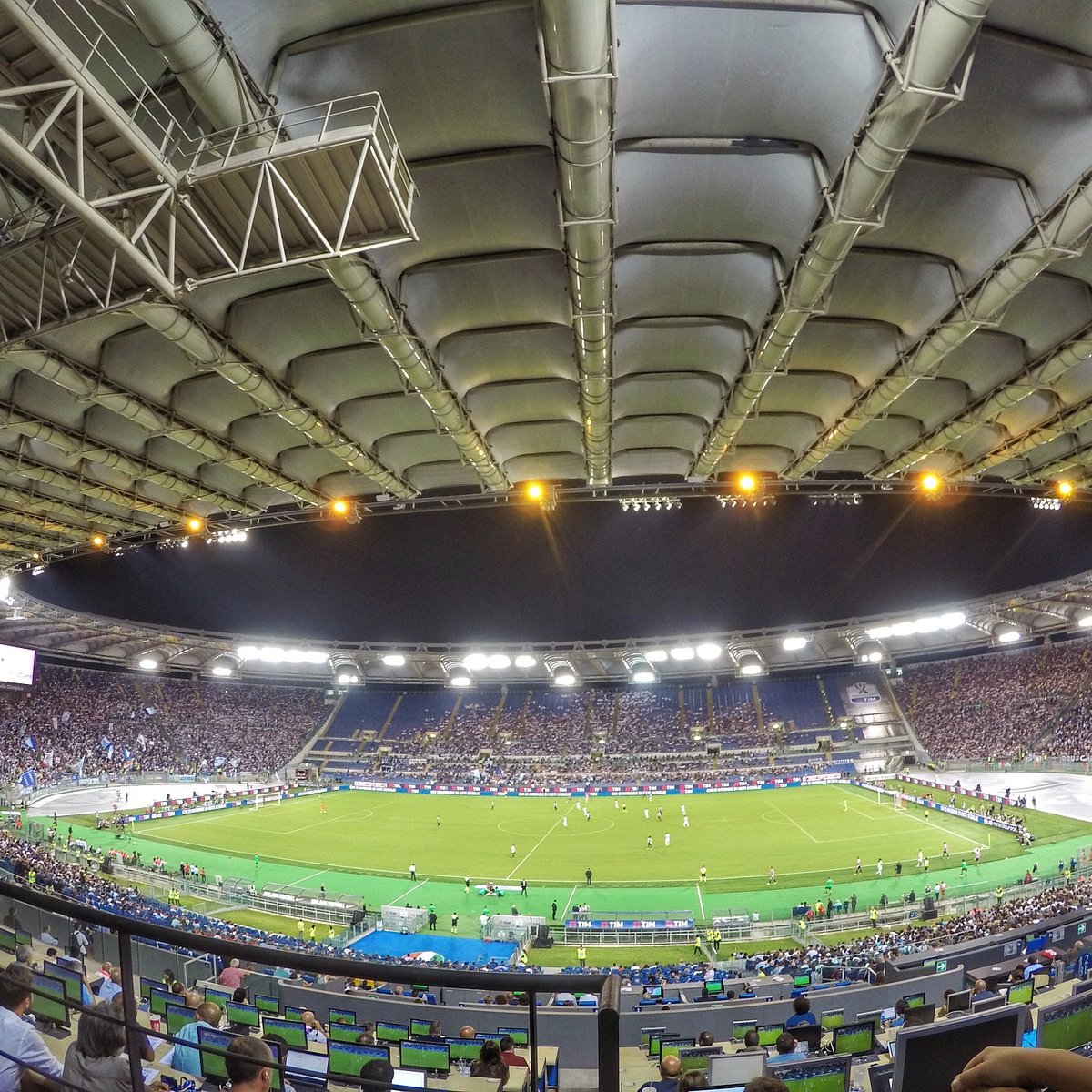The image captures a wide-angle view of a bustling soccer game in a large, bowl-shaped stadium at night. The warm orange and yellow glow of the stadium lights illuminates the scene from above, casting a golden hue over the field and the sea of spectators. The stadium is packed with thousands upon thousands of fans seated in the bleachers, which span from ground level to the upper reaches of the arena. Below, the soccer field is a vivid light green color with darker green edges, dotted with white and blue-clad players engaged in the midst of an active match. The center of the field is occupied by these players, while a running track encircles the field, where individuals can be seen participating in track events. In the foreground of the image, a notable section is occupied by over a hundred people with laptops, likely documenting or streaming the game. The night sky above is clear, indicating a late evening game, possibly around 9 PM. The entire scene is a vibrant tapestry of athletic competition, fan enthusiasm, and the glow of stadium lights.